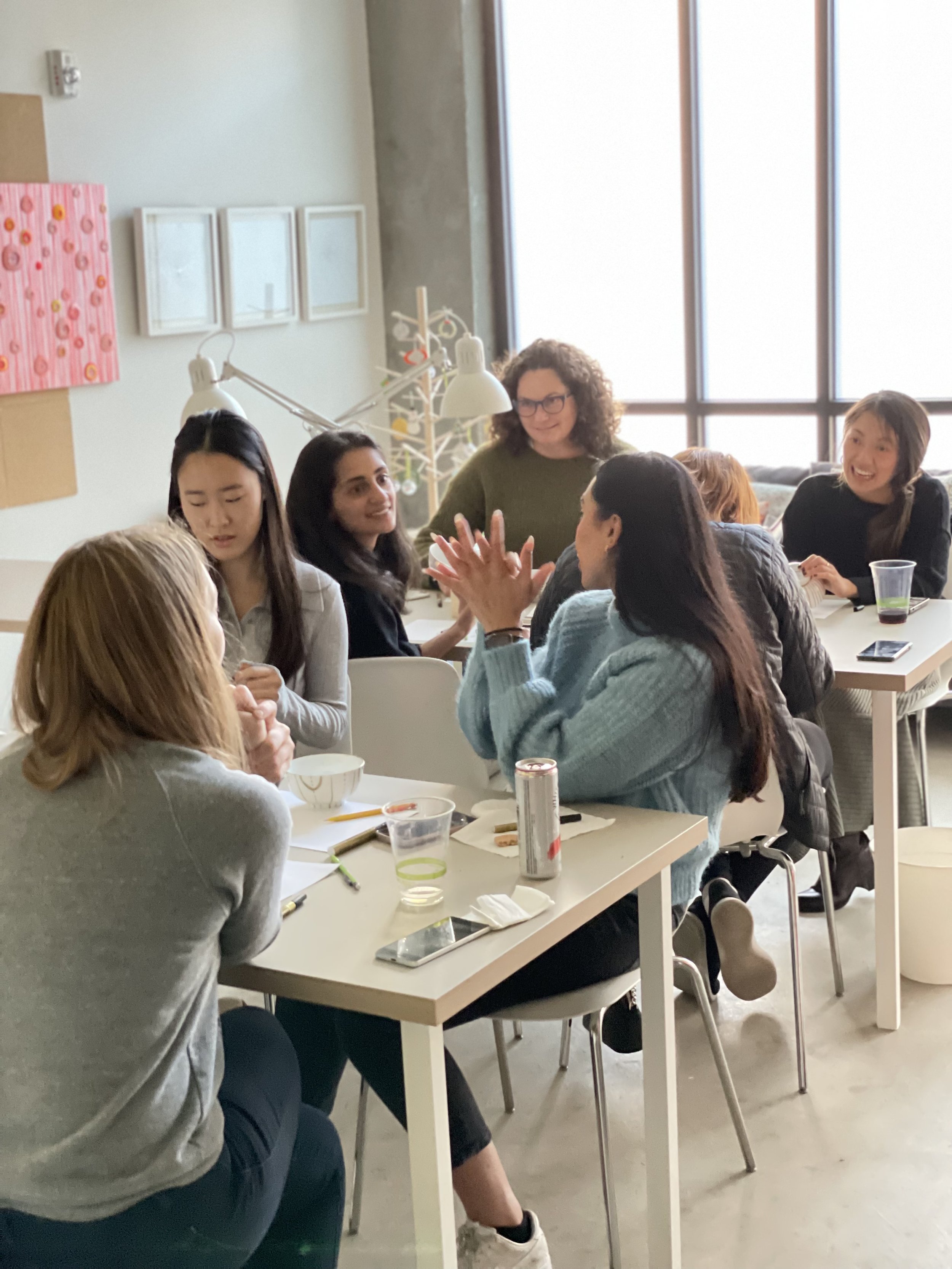The image captures a brightly lit indoor study space during daytime, featuring seven women who are sitting at two white tables. The group includes both white and Asian individuals, mostly appearing young, with one possibly over 40. Three women are seated at the nearest table, and four are at the table further away. The women are engaged in conversations, some facing each other while others turn to speak to different people across the tables. The table surfaces are cluttered with academic materials such as notebooks, papers, pens, alongside mobile phones, drinks in plastic cups and cans, and white bowls. 

The room has white walls and light-colored flooring. Prominent in the background is a large white window allowing bright sunlight to illuminate the space. On the left wall, there's a gray section adorned with decor items, including three picture frames containing paper, a pink object, and a possible cork board. A series of big white lamps hang from the ceiling, further enhancing the room's bright ambiance. The setting, with its emphasis on study materials rather than food, suggests that the women are likely engaged in studying or working together.